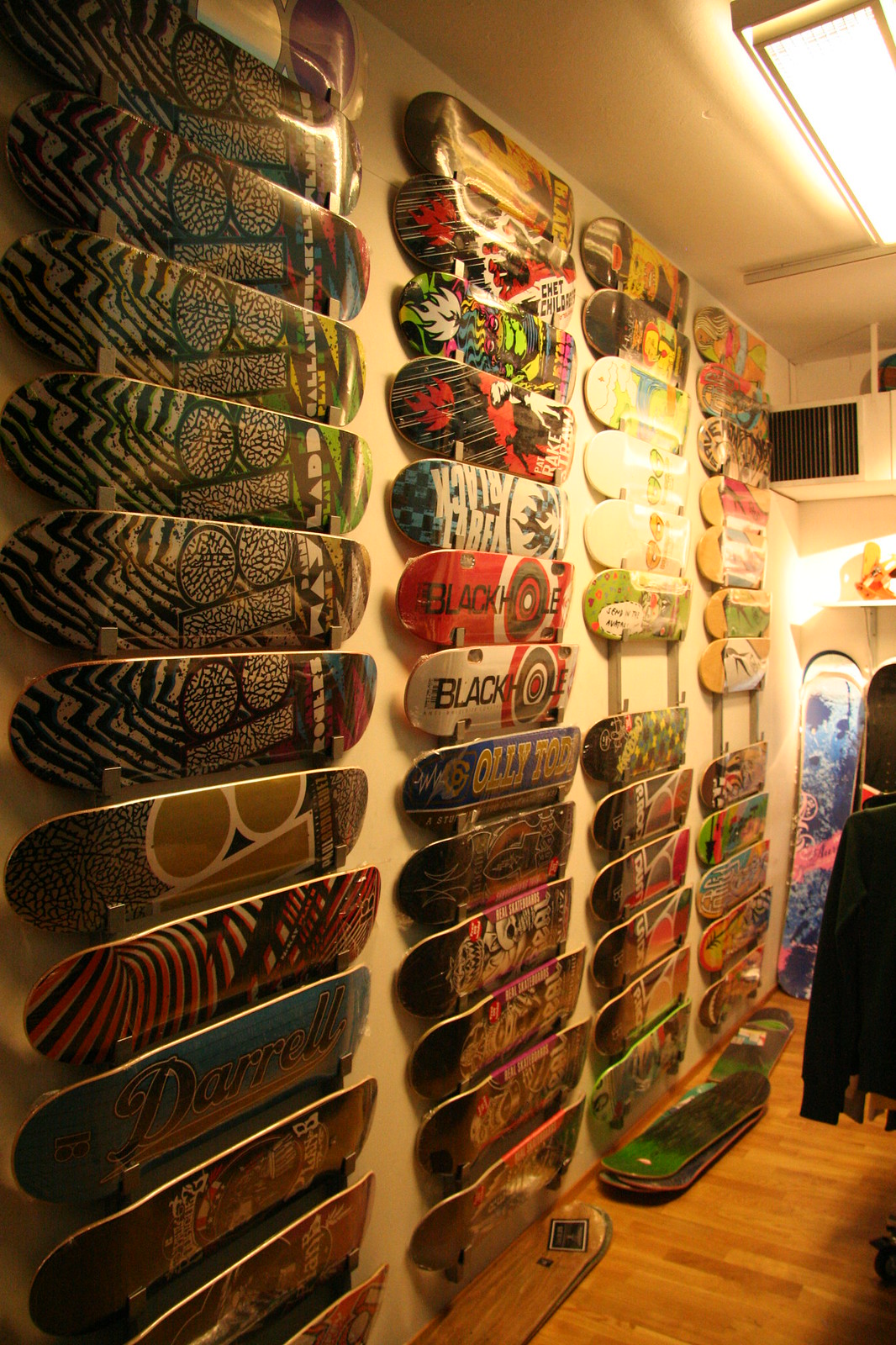The image depicts a detailed and vibrant display wall in a skateboard shop, adorned with numerous skateboard decks. There are four vertical racks extending from the ceiling to the floor, each holding approximately 18-19 decks, all uniformly sized. The decks feature a wide array of colorful patterns and designs, including muted green designs with geometric shapes, blue decks with gold accents, and pink and black swirls. Many decks bear notable names and words such as "Black Hole," "Ollie Todd," and "DARRELL." 

The wall itself is white, allowing the colors of the skateboard decks to pop. There are also several longboards leaning against the wall, not hung up. An air conditioner with a black vent is visible at the top right corner, alongside a large square shop light on the ceiling, illuminating the scene. The bottom of the wall sees additional decks stacked on the ground. Notably, a clothing display is partially visible to the right of the image, indicating the shop's diverse offerings. The detailed setup hints at the shop being not just a retail space but also potentially a repair area or a dedicated collector's showcase.